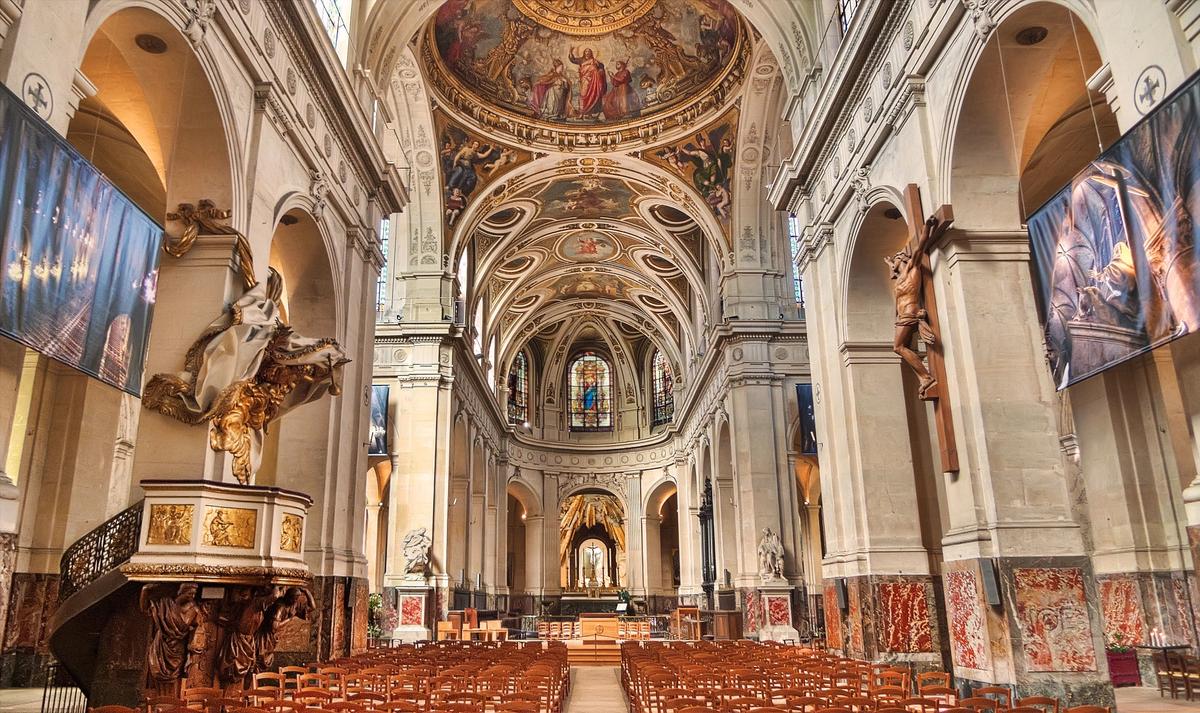This photograph captures the interior of a grand, ornate Roman Catholic cathedral. The first striking feature is the immensely high ceiling adorned with elaborate Renaissance-style murals depicting biblical scenes, centered around a majestic dome. Massive, ancient columns line both sides of the cathedral, featuring intricate floral patterns at their bases and arching peaks that connect them. Gold accents lavishly decorate the various statues and sculptures scattered throughout the space, adding to the overall opulence. In the foreground, there's an array of nearly 100 wooden chairs, all arranged facing a distant lectern where the service is held. A notable, large wooden crucifix hangs prominently from one of the columns, while vivid, stained glass windows illuminate the area with colorful light. Despite its age—which appears to be several centuries—the cathedral also incorporates modern elements, such as large monitors on the sides likely used to aid the congregation's view of proceedings. The combination of detailed biblical art, high ceilings, and extensive seating highlights the cathedral's rich history and grandeur.